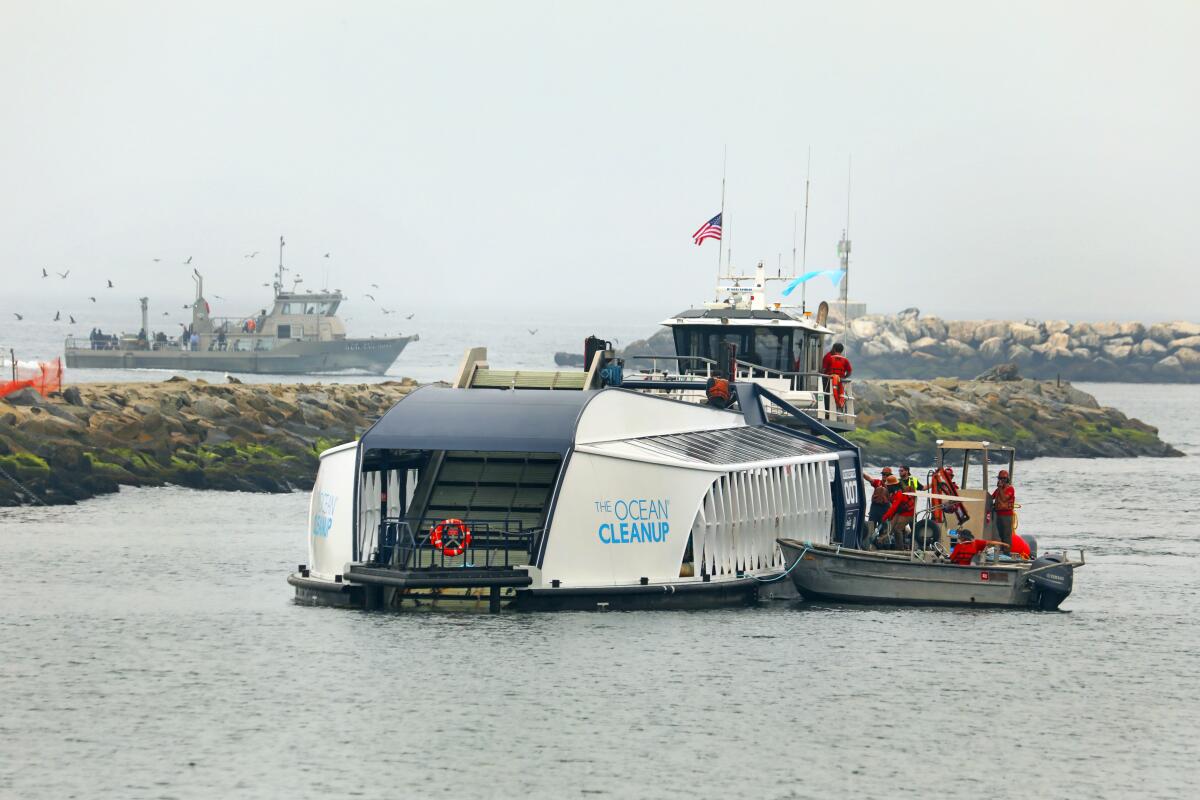In this photograph, a large, modern ship with black and white coloring, bearing the "Ocean Cleanup" label in blue, is prominently featured in the center. The ship flies the USA flag and is accompanied by a smaller motorboat, both carrying people dressed in red uniforms. The scene is set in a blue, tranquil ocean with a clear sky above. To the right of the large ship, two smaller boats are docked, with people in orange or red attire engaged in conversation. The area appears to be within a jetty structure made of rocks, visible in the midground. In the distant background, another sizable boat, possibly a fishing or tourist vessel, is seen amidst a flock of seagulls. The whole atmosphere appears serene but active, with elements of both environmental cleanup and maritime operation present in the image.